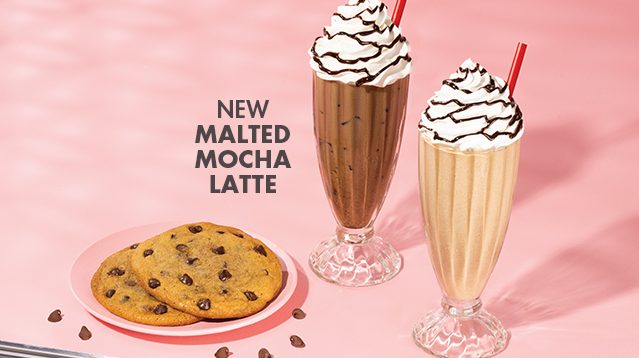The professionally taken photo features a vibrant light pink background that emphasizes the delectable items on display. Central to the composition is a large, round pink plate, adorned with two large, wide chocolate chip cookies, one stacked atop the other. Surrounding the plate are scattered chocolate chips, adding a decorative touch. 

To the right of the plate are two tall, clear glasses resembling classic malt shop milkshake glasses. One glass holds a rich, dark brown milkshake, clearly a chocolate beverage, topped with whipped cream, drizzled with chocolate syrup, and finished with a bright red straw. The other glass contains a light tan milkshake, its creamy beige hue suggesting a vanilla or light chocolate flavor, also garnished similarly with whipped cream, chocolate drizzle, and a red straw.

The dark gray text overlay reads "new malted mocha latte," hinting that these enticing shakes might be part of a new promotional beverage offering. The colors in the image—ranging from light pink, tannish beige, and various shades of chocolate and white—create a warm, inviting atmosphere, perfect for advertising the new malted mocha lattes. While the company name isn't provided, the clarity and arrangement of elements suggest this image is part of a paid advertisement campaign.